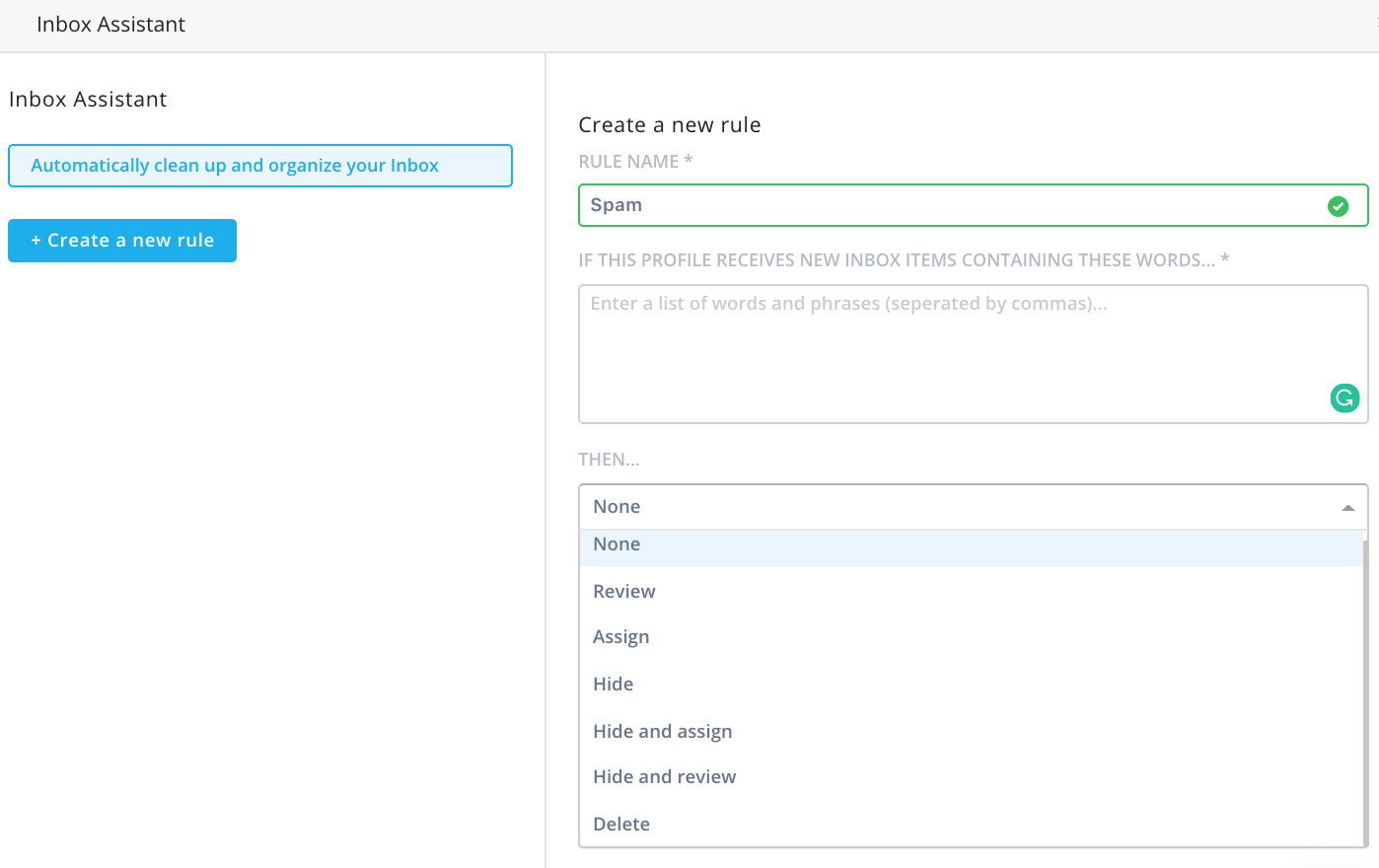This photo captures a screenshot of an "Inbox Assistant," a tool designed for managing emails or work order programs. The image is landscape in orientation, slightly longer than it is tall, and features a gray border across the top, separated by a gray line at the bottom.

On the left side of the screen, starting about a third of the way across the page, a gray vertical line divides the content. To the left of this line, a header reads "Inbox Assistant" followed by a bold blue rectangular box with darker blue text that says, "Automatically Clean Up and Organize Your Inbox." Beneath this, another blue rectangular box with white text and a plus sign prompts, "Create a New Rule." 

On the right side of the border, the phrase "Create a New Rule" appears prominently, with a grayed-out text field labeled "Rule Name" and marked with an asterisk. Below this field, a green rectangular box with the word "Spam" in black text sits next to a green circle containing a white checkmark. This is followed by an instruction that reads, "If this profile receives new inbox items containing these words," accompanied by a text entry box for input.

Further down, a header labeled "Then" introduces a gray box presenting various options, including "None," "Review," "Assign," "Hide," "Hide and Assign," "Hide and Review," and "Delete." These options indicate the actions to be taken based on the specified rule criteria.